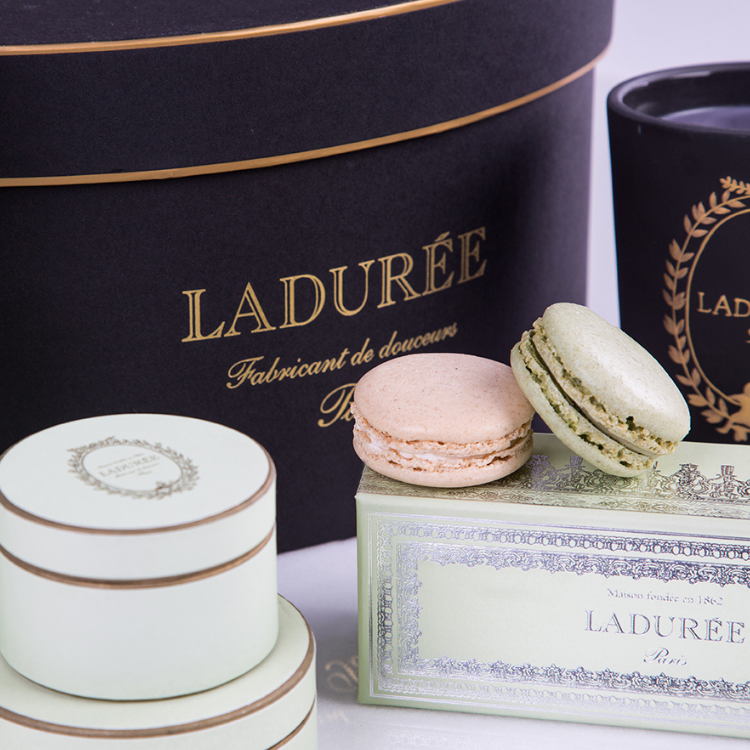The image showcases a collection of elegantly packaged products, prominently featuring Ladurée's luxury confectionery items and containers. At the center, two macarons take the spotlight: a pink one with cream filling, accompanied by a green macaron with matching green filling, both resting atop a pastel green box adorned with intricate black etchings. The box is labeled "LADURÉE" in gold lettering, followed by the phrase "Fabricant de Douceurs" in cursive, affirming the French origin of these sweets. 

To the left of the macarons, there's a stack of circular boxes in muted tones, with brown detailing, the smaller box perched atop a slightly larger one. In the background, a larger, blue cylindrical container, possibly made of paper or cardboard, also bears the Ladurée branding in gold, along with the same French inscription. 

On the lower right, the scene includes a black coffee mug accented with gold grain designs and partially visible letters "LAD." The upper right corner reveals part of an ornate, leaf-patterned item resembling a candle holder, enhancing the overall luxurious aesthetic of the collection.